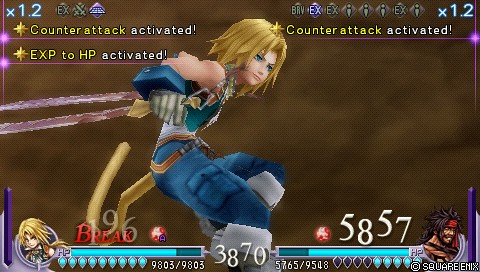In this screenshot from a video game, a character with long blonde hair, clad in blue pants and a white top, stands poised for battle. The character, who has a masculine build with muscular arms, wields a sword in one hand and wears impressive gloves that enhance their fighting prowess. The game's interface displays the message "Counter-Attack Activated" and "Experience 2 HP Activated x1.2," signaling the execution of special abilities. Additionally, indicators of "58" and "57" with the word "Break" appear in the lower corner of the screen, suggesting a timed challenge or countdown. The backdrop is a rich brown, setting the stage for what appears to be a dynamic and intense fighting game scene.